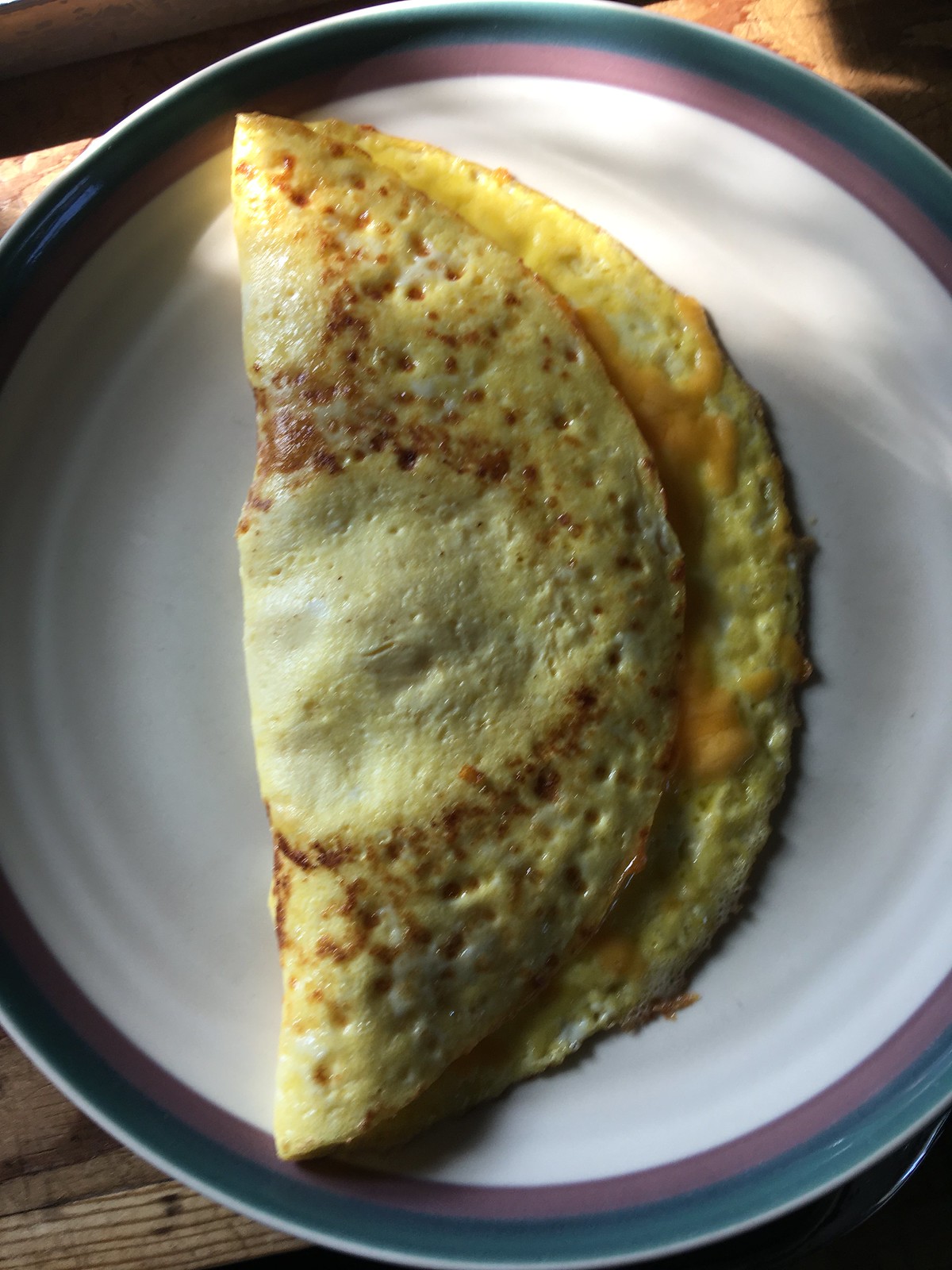The photograph is a detailed close-up of an omelette on a ceramic plate, captured in portrait orientation while looking straight down. The plate, partially visible, features a white center with ridges around the circumference, followed by a decorative edge composed of a mauve band, a greenish turquoise stripe, and an outer white band. The omelette, yellow with brown and golden hues indicating some overcooking, is folded in half, slightly off-center to the left. Dark red Leicester-style cheese oozes from the fold, and the surface of the omelette shows dimples created during cooking. The plate rests on a light brown table, with a portion of a wooden floor visible in the right-hand corner of the image.